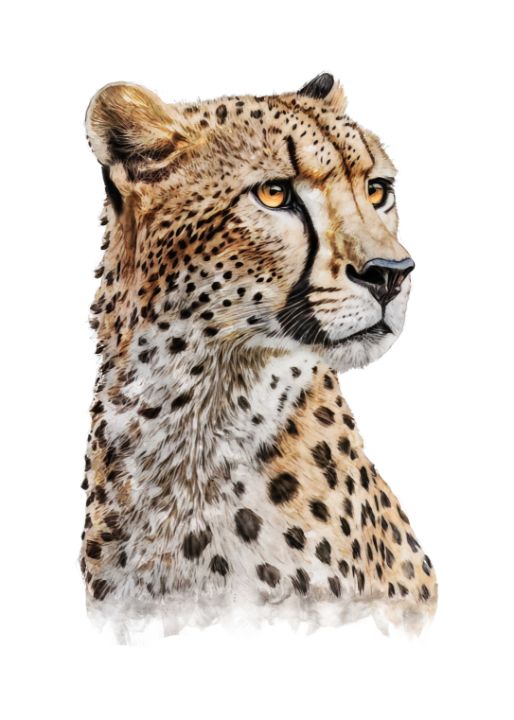This is a meticulously hand-drawn image of a cheetah, depicted using what appears to be colored pencils or watercolors. The cheetah is set against a completely white background, which provides no context or reference to its surroundings. The image focuses on the cheetah's head and part of its neck, terminating around the chest area in a delicate, feathery fashion typical of watercolor techniques.

The cheetah sports predominantly brown fur, flecked with distinct black and gray spots. Its rounded ears are brownish, and it has a striking black nose. Around its mouth, fine white hairs are visible, lending a detailed realism to the drawing. The cheetah's eyes are a vibrant yellow, intently gazing to the right, conveying a composed yet alert expression. The spotting pattern differs with smaller spots concentrated on its head and larger ones appearing on its chest area, where the white fur interspersed with the spots almost forms faint stripes.

The overall presentation of the cheetah exudes a sense of serene vigilance, with the detailed and delicate coloring highlighting the artist's skill and attention to realism.